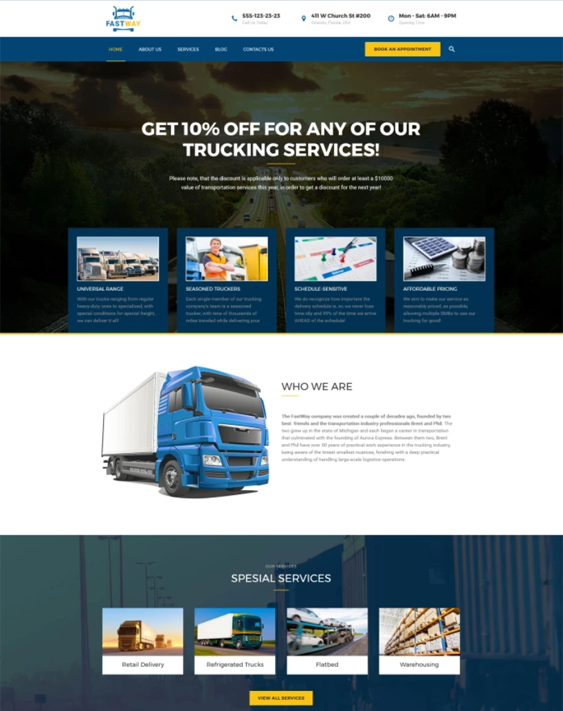The image appears to be a screenshot of a trucking company's website, featuring a detailed and visually structured layout. The background of both the top and bottom halves is filled with a faded blue overlay, with the top showcasing a picture of a highway and the bottom depicting a storage area. Centered in the middle is a white space displaying an image of a truck. Above this space is a prominent banner that reads "Get 10% off for any of our trucking services" in white text.

Below the banner is some smaller, less legible text. Directly beneath this are four interactive icons from left to right: the first is an image of trucks, the second shows a person wearing an orange safety vest and looking at the camera, the third is an illustration of a calendar with colorful pins (red, blue, and green), and the fourth displays a calculator, a pen, and some dimes.

Furthermore, there is a section featuring special services each represented by different images and captions: "Detail Delivery" with a picture of a truck, "Refrigerated Trucks," "Flatbed," and "Warehousing." The "Who We Are" section includes a description of the company, though the specifics of the text are not detailed here. The overall design of the website appears well-organized, providing clear and engaging visual information about the company's offerings and services.